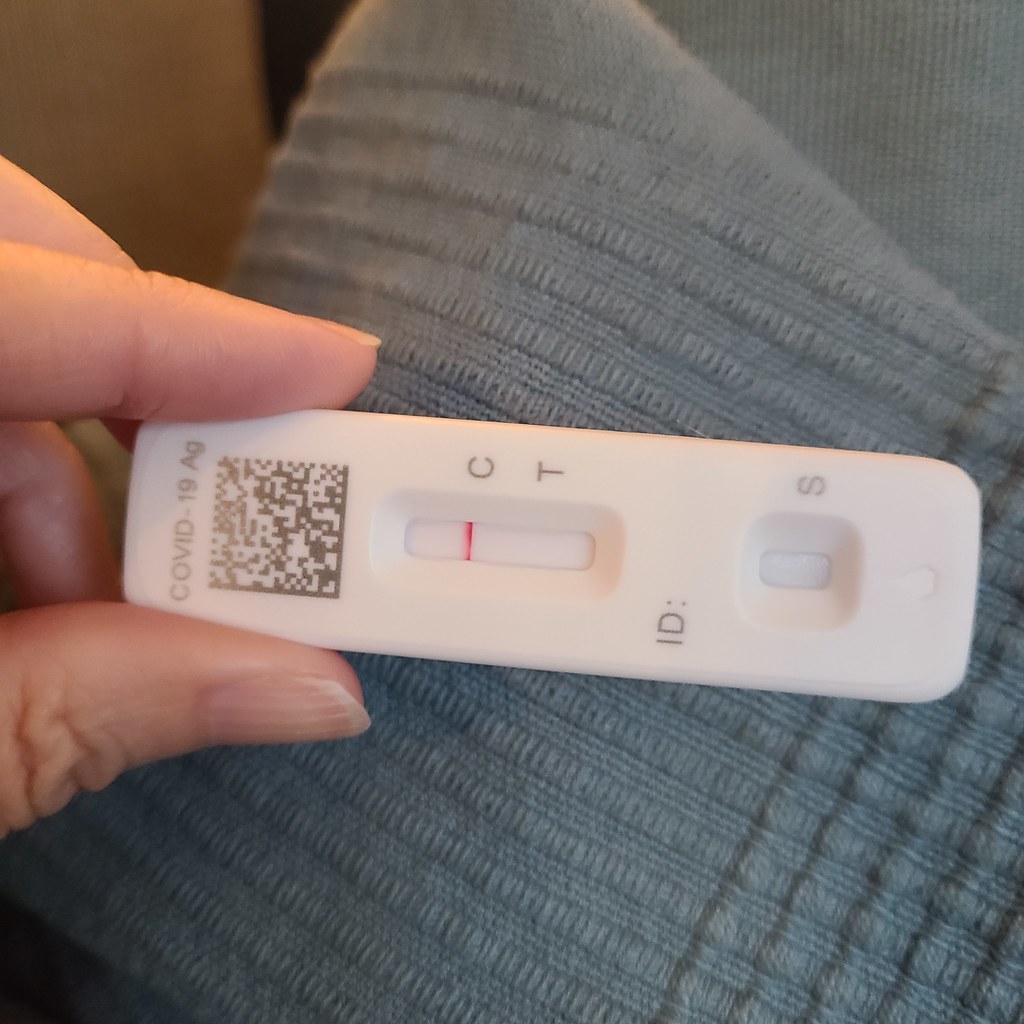A detailed caption for the image could be:

"A close-up photograph of a portable COVID-19 antigen test pen, held in a large hand with the index finger resting on top and the thumb at the bottom. The pen itself is a small rectangular device with various features prominently displayed. On the left side, the label 'COVID-19 AG' is clearly visible. Beneath this label, there is a black QR code consisting of a pattern of white and black squares.

In the center of the test pen is a rectangular opening. At the top of this opening, the letters 'C' and 'T' are inscribed. Directly below the 'T,' there is a distinctive dark red line. The lower half of the device features the letters 'I' and 'D' separated by a dash, followed by another smaller rectangular opening that is empty. Additionally, the letter 'S' is marked on the side of the test pen.

The entire test pen is white with black inscriptions. The background of the image appears to be a cloth material, possibly a towel, characterized by a blue-green hue with linear patterns."